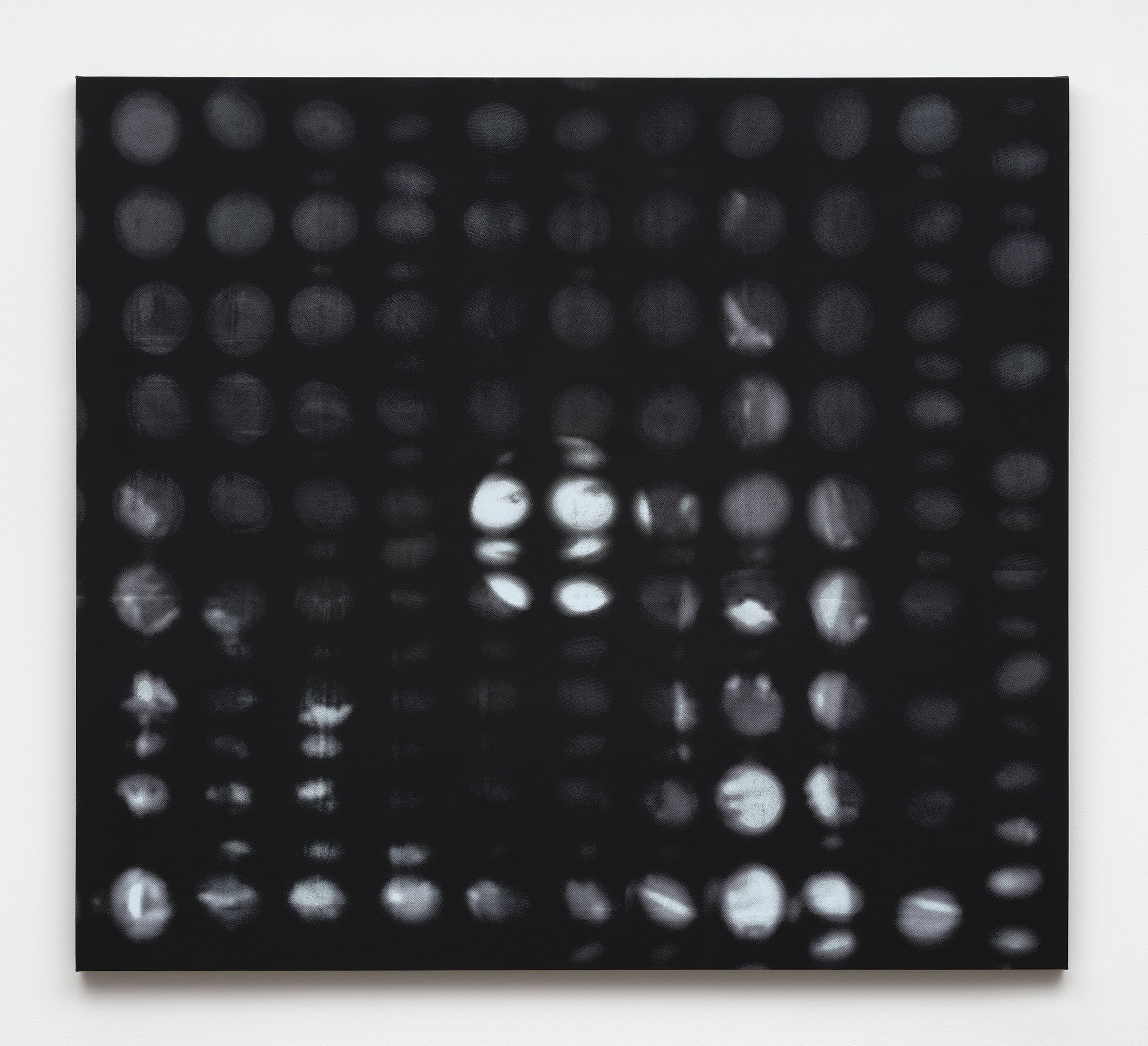This black-and-white photograph appears to be taken through a grate or screen featuring a grid pattern of circular cutouts. The overall shape is nearly square, with a cream-colored outer border that transitions into a black interior filled with these evenly spaced circles. The image beyond the grate is abstract and blurry, presenting a stark contrast between light and darkness. In the center of the image, a prominent bright white circle, resembling a globe or moon, draws attention. Adjacent to this central circle, there are additional white silhouettes and light patches, creating an enigmatic and thought-provoking scene. The bottom half of the image features a white band stretching across the width, contributing to the digital, almost Photoshopped aesthetic, with a vague drop shadow effect emphasizing the image’s abstract nature.